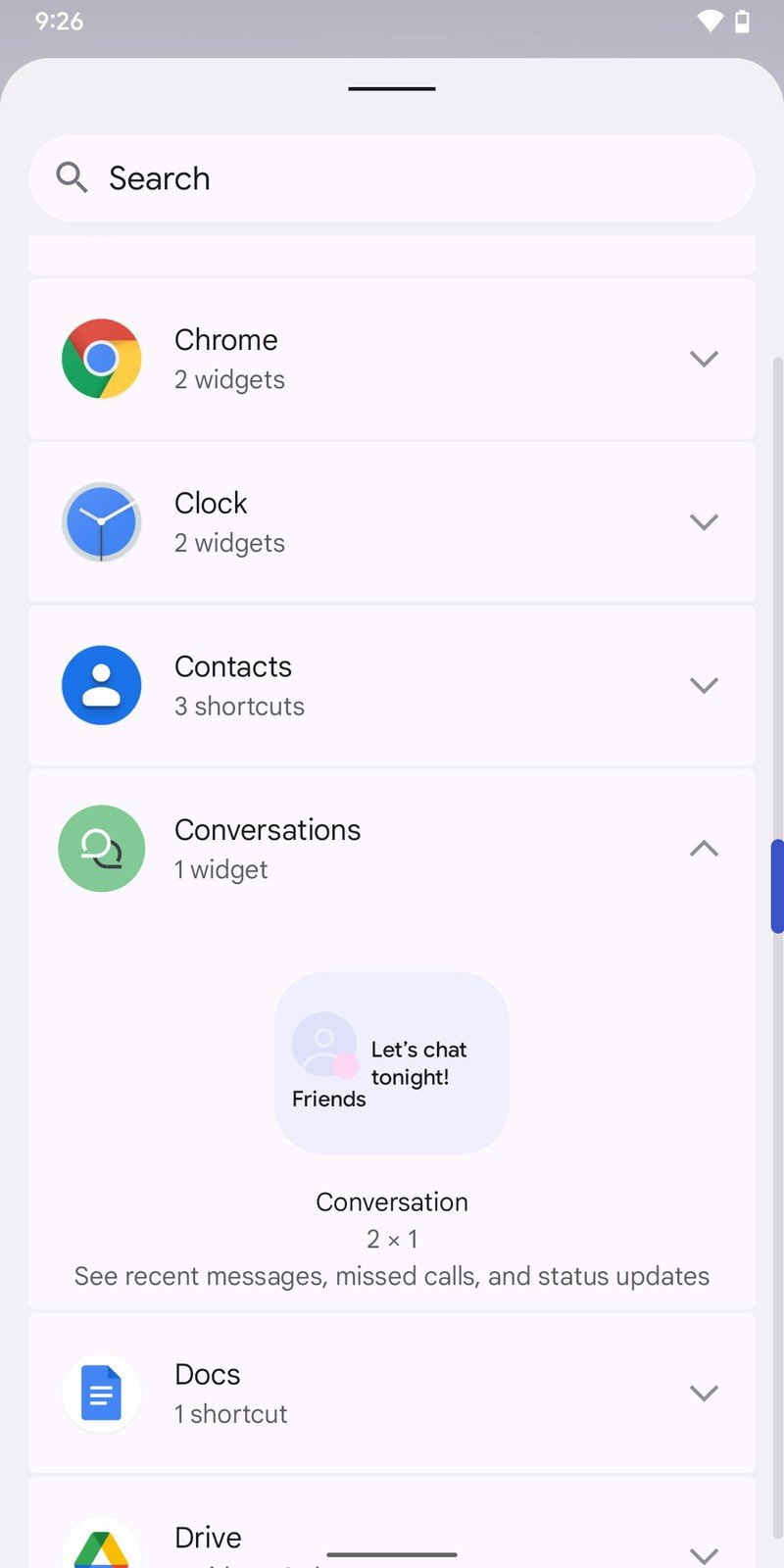The image is a screenshot of an Android phone, potentially a Google device, displaying an infographic in a list format. At the top of the image is a search bar. Below the search bar, the list shows several entries, each accompanied by their respective icons and expandable down arrows for more detail. 

1. **Chrome**:
    - Icon: Google Chrome symbol.
    - Description: "2 widgets."
    - Arrow: Indicating expandable details.

2. **Clock**:
    - Icon: An image of a clock with white hands.
    - Description: "2 widgets."
    - Arrow: Indicating expandable details.

3. **Contacts**:
    - Icon: A blue circle with a small white dot and a medium-sized white dot, resembling a head and shoulders.
    - Description: "3 shortcuts."
    - Arrow: Indicating expandable details.

4. **Conversations** (expanded):
    - Icon: A circular icon.
    - Description: "1 widget."
    - Details: Displayed as a 2x1 widget showing recent messages, missed calls, and status updates. The widget reads "Conversation: Let's chat tonight," and is labeled "Friends."

5. **Docs**:
    - Icon: Not detailed in description.
    - Description: "1 shortcut."
    - Arrow: Indicating expandable details (not expanded).

6. **Drive**:
    - Icon: Not detailed in description.
    - Description: Included in the list but no specific details provided.

In summary, the image highlights a list of applications on an Android device, each with widget and shortcut options, some of which are expandable for more details.